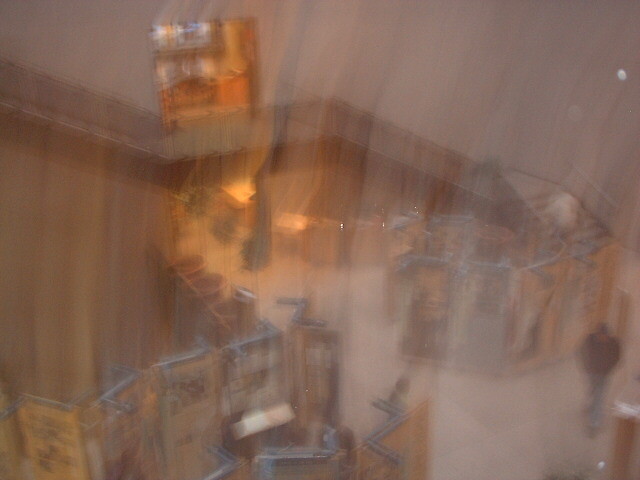This image showcases a highly blurred scene, reminiscent of a video game environment, characterized by vertical and horizontal motion streaks. Starting from the top left corner, there's a distinct roof structure or overhang, which appears brown and follows a path that turns several times before tapering off. Below this roofline, a wall is partially visible. In the bottom left, there is a protruding panel, which transitions into three additional panels, forming a sequence. A square, house-like structure painted in yellow occupies a central position in the scene. To the right of this structure, a tree is discernible amidst the blur. Adding a dynamic element to the image, a person is seen walking, contributing to the overall sense of movement.